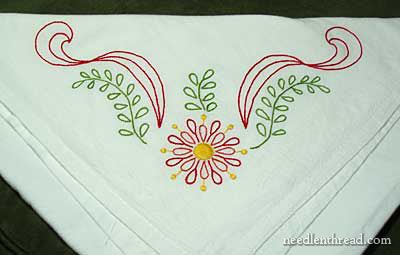The image showcases a white handkerchief elegantly folded into a triangle, displaying intricate embroidery. The design, dominated by vibrant shades of red, green, and yellow, features a central red flower with a yellow center and tips, akin to a daisy. Surrounding the flower are stylized leaves, forming a vine pattern, extending upward on both sides of the central motif. These vines, embroidered in red, weave into swirling designs along the outer edges, accentuated by green leaves. Completing the detailed artwork, the design includes additional mini vine patterns strategically placed above the flower. The handkerchief, highlighted against a white background, also includes a subtle reference to a website, needleandthread.com, stitched in the corner, further emphasizing its artisanal craftsmanship.